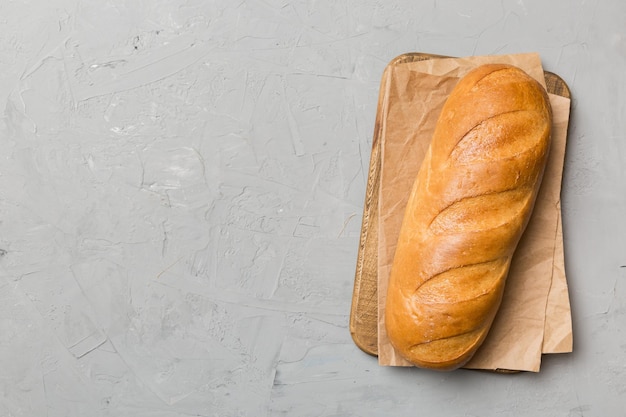The image depicts a long, oval-shaped toasted baguette with a light brown, yellowish hue, resting on a folded brown sheet of paper. This paper is placed on a rectangular wooden serving board with a distinct beveled edge. The board, showcasing a natural wood grain, contrasts with the white surface beneath it, which has noticeable black stains and artistic markings. The white platform underneath exhibits a gray, spackled texture with a slight shine on the left side. The baguette features five elongated oval indentations across its top.